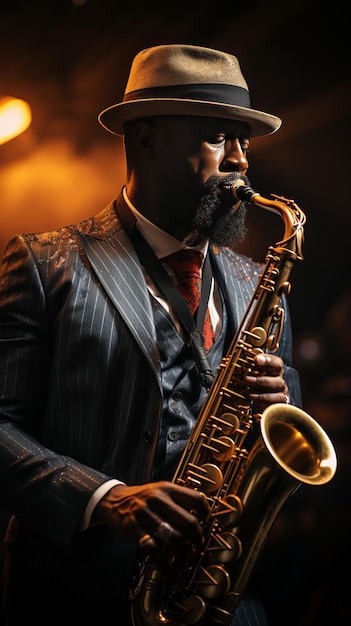This image portrays a dark-skinned black man immersed in playing a gleaming copper-tone saxophone. He sports a tan fedora hat with a black band, complementing his full black beard and mustache. Dressed in a sophisticated dark gray pinstripe suit with a matching waistcoat, a pristine white shirt, and a deep wine-red tie, he exudes a classic jazz vibe. His right hand, adorned with two rings, grips the saxophone with practiced ease. Suspended from his neck by a strap, the saxophone suggests both movement and stability. The background is a blurred gradient of dark and orange hues, faintly illuminating the scene and highlighting the musician, possibly indicating an indoor setting bathed in dim, moody light.